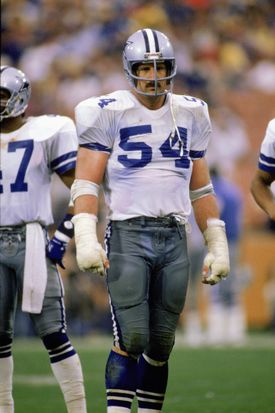This is a tall rectangular photograph of a Dallas Cowboys football player, visible from his ankles up, standing on the green field. His body is facing forward. He is wearing a somewhat dirty white jersey with the blue number 54 on the front and shoulders, along with dark grayish-blue pants featuring a white and dark blue stripe down the sides. The pants are skin tight with visible padding, and he is also wearing dark blue socks with multiple white horizontal lines. His arms are flared out, showing white, somewhat dirty casts on both hands and additional white cloth wrapped around his elbows. He has a silver helmet with a face mask and a light blue stripe bordered by navy blue stripes running across it. To his left stands another player, similarly outfitted, with black skin, the digit seven visible on his jersey, and a white towel hanging from his waist over his left leg. The background reveals a blurred audience of spectators, emphasizing the stadium setting, while no opposition players can be seen in the photo. Additionally, a right hand clad in a uniform enters the frame from the center, suggesting another nearby presence.